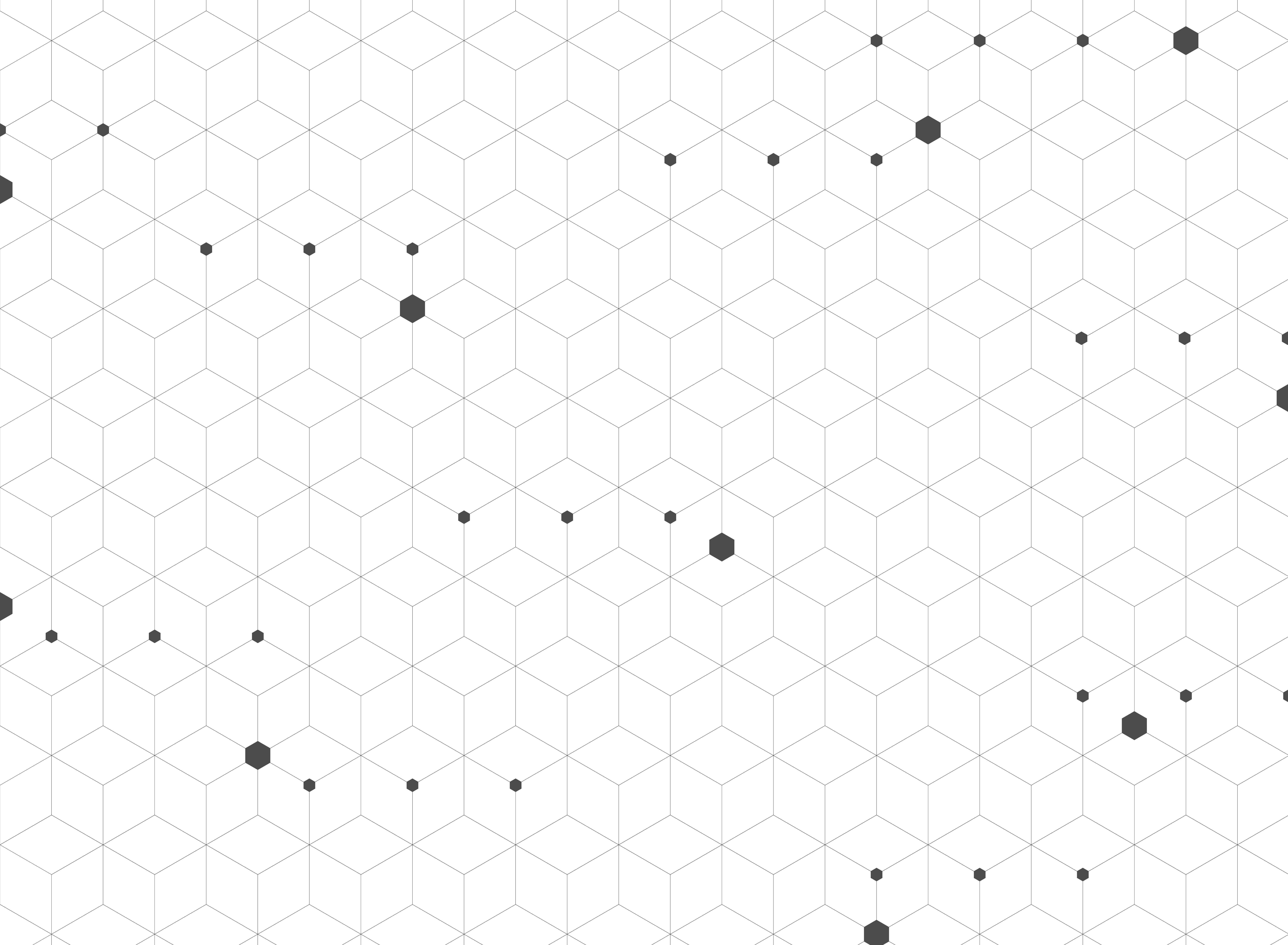The image showcases a detailed design on a rectangular-shaped screen, featuring intricate patterns and shapes. The primary design element consists of interlocking cuboid-like 3D patterns, entirely drawn in shades of gray. These patterns are composed of illuminated lines that form the structure of the cubes. Within the design, various hexagonal spots are randomly distributed, adding depth and variation to the artwork. The hexagons, which vary in size, are a darker shade of gray compared to the rest of the design, and are strategically placed along the corners and edges of the cuboid shapes. The combination of 3D cubes and hexagonal accents results in a captivating and visually striking composition.